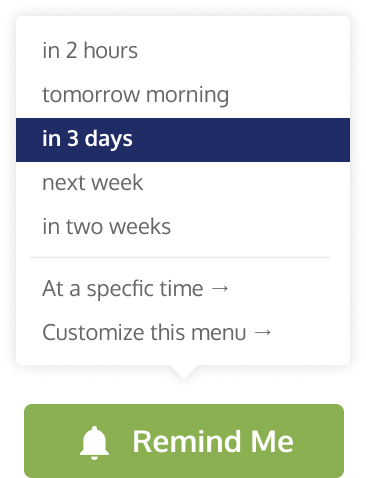The image features a vertically aligned menu set against a white background, designed in the shape of a speech bubble that tapers downward. The menu presents several scheduling options, each separated by a line. The options listed are as follows:
1. In two hours
2. Tomorrow morning
3. In three days
4. Next week
5. In two weeks

Below this list, an instruction reads, "At a specific time," accompanied by an arrow pointing to the right. Adjacent to this is another instruction, "Customize this menu," also with a rightward arrow. 

Beneath the options section, there is a prominent green button labeled "Remind me," with the text "Remind me" written in white. To the left of this button is an alarm bell icon, indicating the nature of a reminder or notification system.

The overall design is simple yet functional, focusing on usability with clearly defined options for setting reminders.